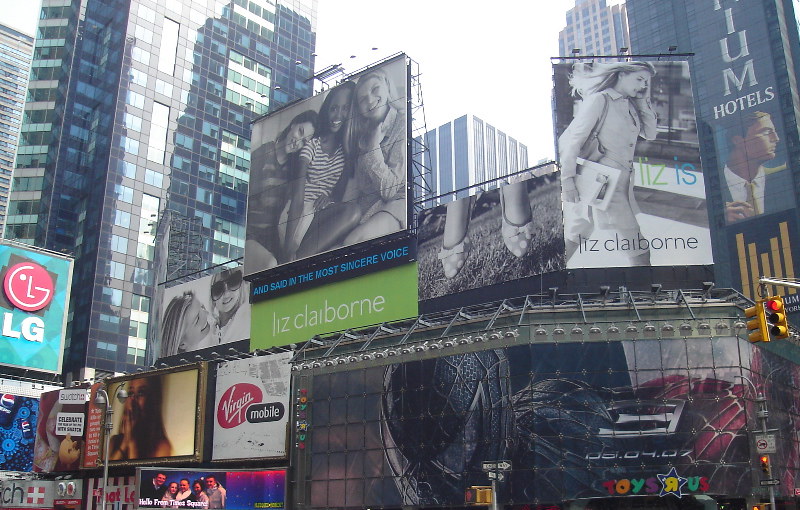This vibrant image captures the bustling downtown area teeming with activity and commercial signage. Prominent storefronts and billboards dominate the scene, including recognizable brands like Toys R Us, Virgin Mobile, and LG. The towering buildings, primarily colored in shades of black with dark blue windows, contrast strikingly against a solitary light medium brown structure. Street lights add to the urban atmosphere, while numerous billboards display various advertisements.

One notable billboard features an advertisement for Liz Claiborne, showcasing a professional woman striding purposefully with a phone in one hand and a couple of papers in the other. Another Liz Claiborne sign depicts three women, likely friends, comfortably sitting and engaging in conversation, enjoying each other’s company. Additionally, another billboard shows two women smiling warmly at each other, exuding a sense of camaraderie and happiness. The scene is a quintessential representation of urban life, encapsulated by the hustle, advertising, and social interactions.